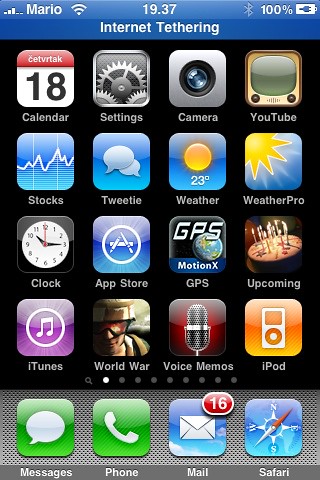The image depicts a detailed and vibrant screenshot of an iPhone home screen in portrait orientation. At the top, the status bar includes various indicators: "Mario" is displayed in white on the left, suggesting the device owner's name, followed by a Wi-Fi signal indication, time set at 19:37, a Bluetooth icon, and a fully charged battery shown at 100%. The phrase "Internet Tethering" is prominently featured in a blue horizontal band.

The home screen showcases an array of 18 app icons, each distinctively colorful against a black background. The apps include Calendar, Settings, Camera, YouTube, Stocks, Tweety, Weather, Weather Pro, Clock, App Store, GPS, Upcoming, iTunes, World War, Voice Memos, and iPod. Below these icons, there is a gold horizontal band containing the navigation buttons, consisting of Messages, Phone, Mail (indicating 16 unread emails), and Safari.

Overall, the screenshot reflects a typical iOS interface, blending illustrated icons with sleek graphic design. The image is crisp and clear, emphasizing the vivid colors—various shades of gray, green, white, blue, orange, red, maroon, and purple. The well-lit and bright setting makes it easy to distinguish and read all elements on the screen.